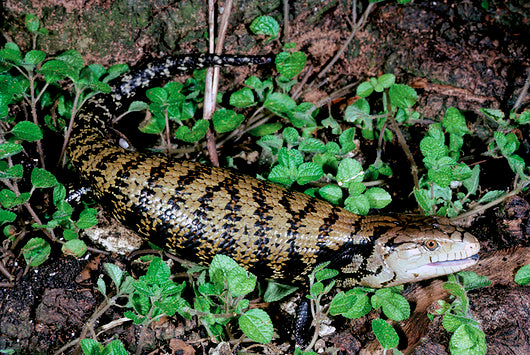This color photo captures a large, fat lizard resembling an iguana, situated outdoors on a muddy or soiled ground, surrounded by various low-to-the-ground plants and clovers, suggesting a forest bed or an unkempt garden area. The lizard's head, which has a snake-like appearance, is positioned in the lower right corner of the image, with its yellow eyes and black pupils gazing to the right. Its mouth is slightly open, revealing a whitish underside of its face. The lizard's body, curving around to its tail in the top center of the photo, features a scaly texture with a grayish-green base color interspersed with a striking pattern of black scales. Its back is adorned with approximately 10 to 20 vertical stripes, each containing a small orange spot, which become thicker near the tail until the tail itself turns completely black. The background is a mix of green ivy vine, brown twigs, mud, and other vegetation, accentuating the lizard's significant and active presence in its natural habitat.